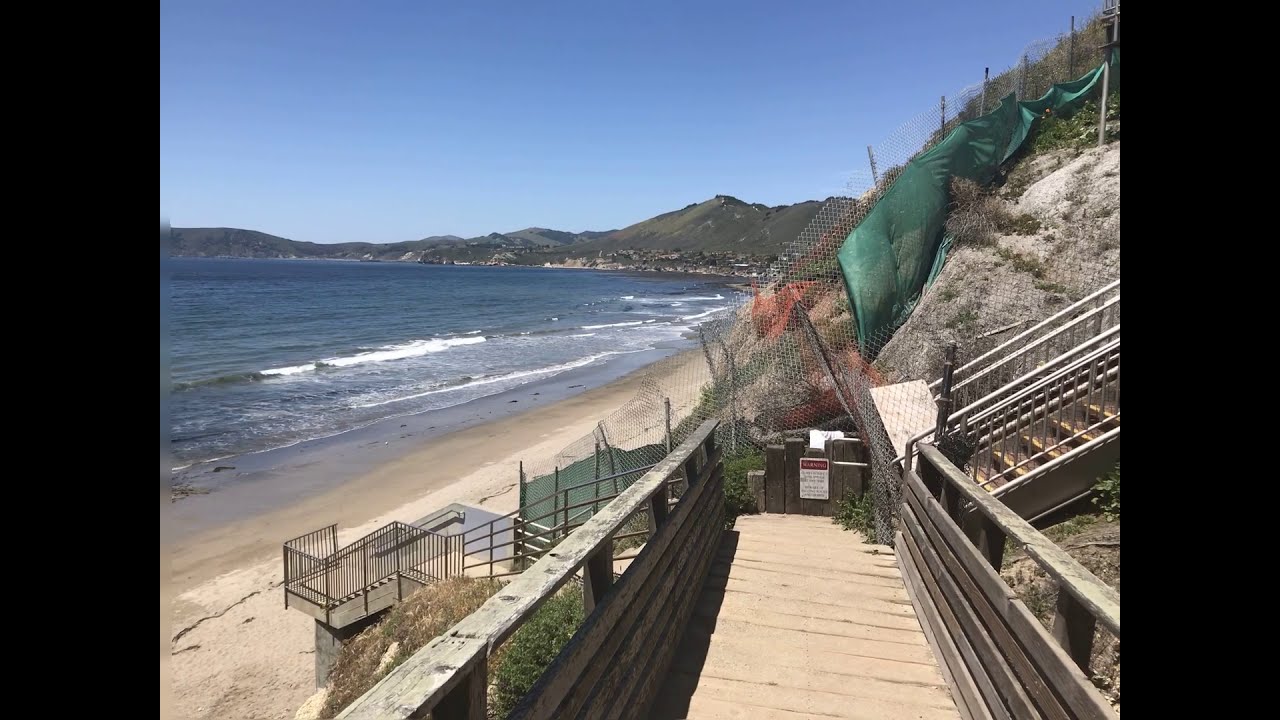The photograph captures a serene, deserted beach scene taken from an elevated wooden boardwalk. The boardwalk runs through the foreground and stretches into the distance, where it eventually connects to a set of stairs. These stairs descend towards the sandy beach, aligning with a green cloth or mesh fence on the right-hand side of the image. The clear blue ocean ahead displays white-capped waves as they crash against the light beige sand. In the background, low mountains rise against a flawless blue sky, offering a picturesque backdrop. The beach is entirely empty, emphasizing the tranquility of the setting. The overall composition is bordered by a thick black edge on both the left and right sides of the photograph, adding a frame-like effect to the peaceful coastal landscape.